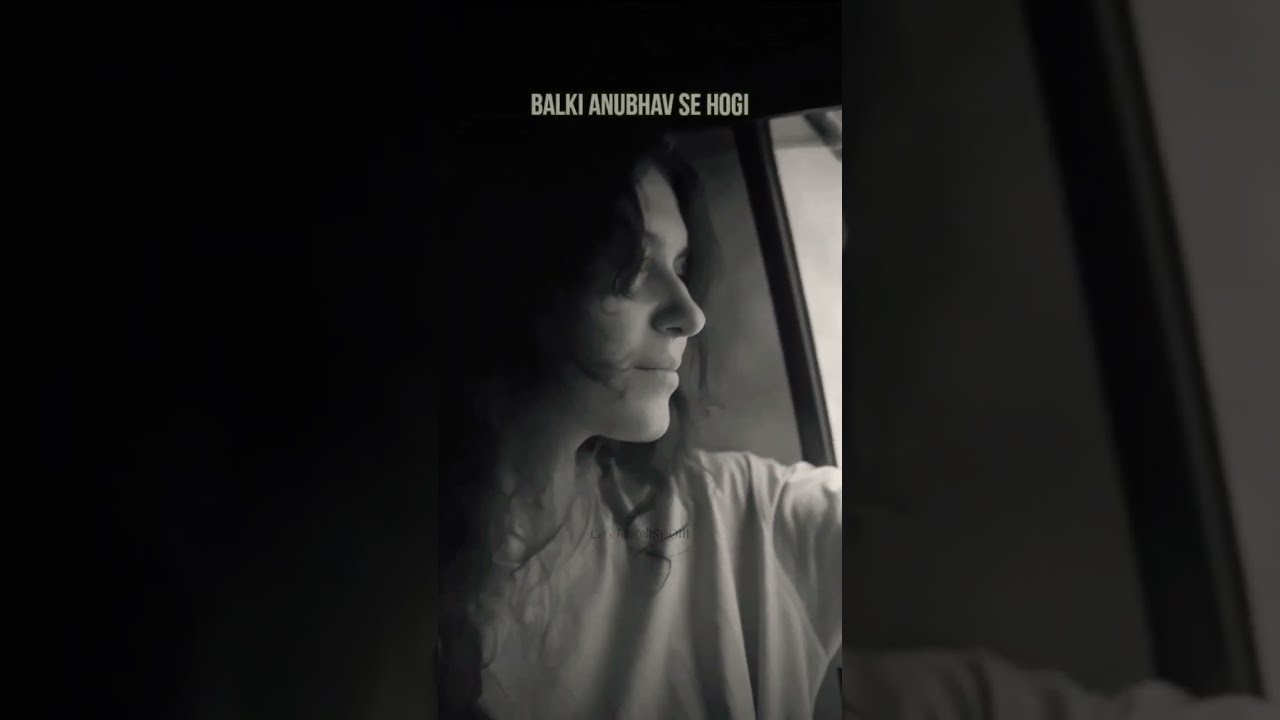The image is a black and white, high-definition TV-shaped composition divided into three segments, focusing primarily on the central photograph. The central segment features a woman with long, slightly wavy black hair, wearing a loose white t-shirt. She is seated in the back of a car, looking to her left and out the window. Her expression appears to be a subtle smile as strands of her hair partly cover her face. Above her image, in bold white text, the title "BALKI ANUBHAV S. HOGI" is written in all capital letters. Flanking this main photograph, the left and right segments are darker and partially faded close-ups of the central image, serving as a border. The left side is indistinct and almost black, while the right side shows part of her arm and the car window. This artsy photograph has a bright light source coming from the upper right corner, enhancing the contrast with the darker surrounding areas.